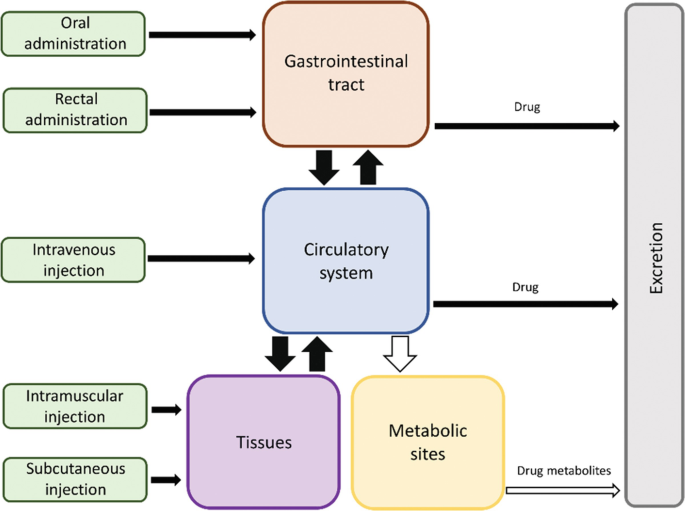The image is a detailed diagram illustrating the pathways of medication administration and their journey within the body. On the left side, there are long rectangles labeled "oral administration" and "rectal administration," both directing with arrows to a large tan square labeled "gastrointestinal tract." The gastrointestinal tract connects via arrows to the "circulatory system," which is a central node in the diagram. Additionally, "intravenous injection" is shown with an arrow leading directly to the circulatory system, while "intramuscular injection" and "subcutaneous injection" lead to a large purple square labeled "tissues." The tissues connect to "metabolic sites," and ultimately everything converges to a vertical gray rectangle labeled "excretion" which represents the endpoint of drug metabolism and elimination from the body. Each step is depicted with clear connections between each administration method, the body systems involved (gastrointestinal tract, circulatory system, tissues, metabolic sites), and the final excretion of drug metabolites.